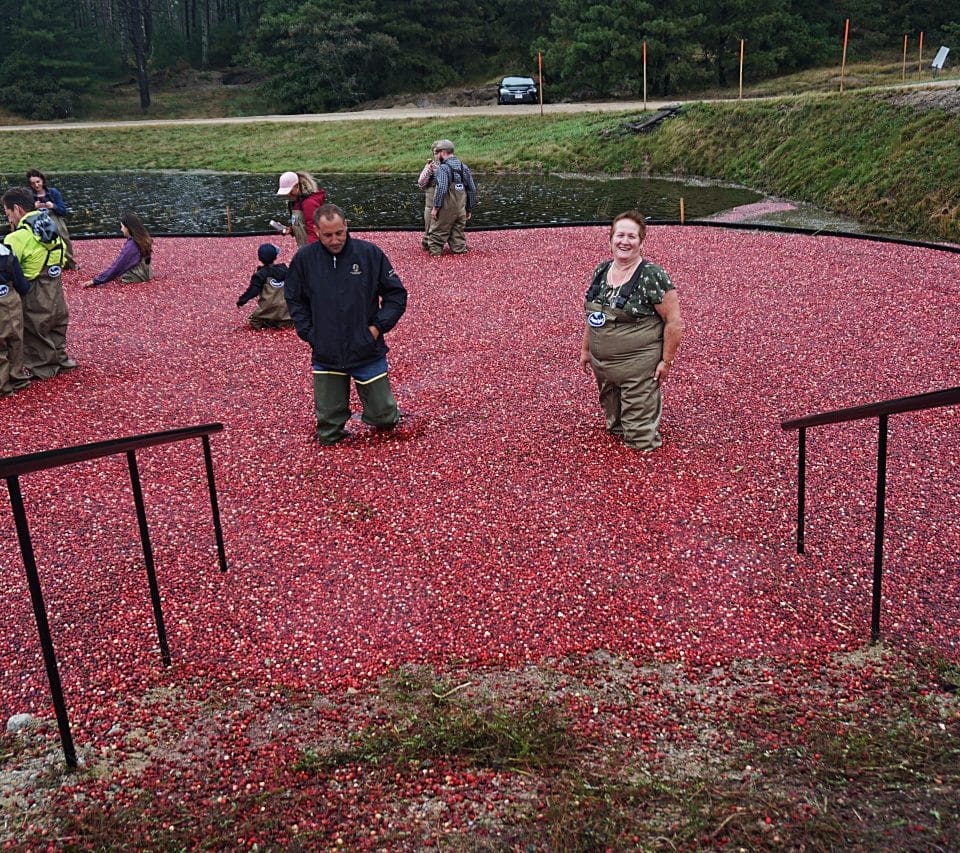In this outdoor photograph captured on a dimly lit day, a group of people are seen standing in what appears to be an emptied swimming pool that has now been filled with what looks like an abundance of red fruits, possibly grapes. The individuals are clad in waders, suggesting that they are engaging in an activity involving the red fruits, likely treading or crushing them with their legs. The background of the image features a lush green landscape, accentuated by a forest of trees, adding a natural contrast to the vivid red fruits in the foreground.